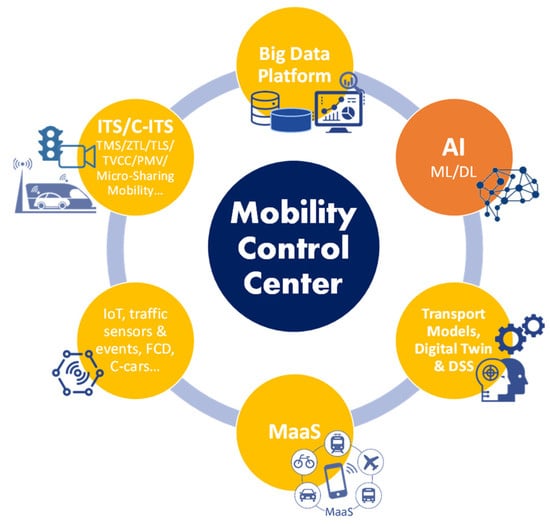The image depicts a detailed diagram representing the structure and components of a Mobility Control Center model, centralized around a dark blue circular core labeled in white text as "Mobility Control Center." Radiating from this central circle, a light blue ring encompasses six evenly spaced sections, each enclosed in either a yellow or orange circle and adorned with illustrative icons reflecting their respective functions. 

Starting from the top and moving clockwise, the first section labeled "Big Data Platform" features an image resembling computer equipment and storage cylinders, emphasizing data infrastructure. Next, an orange circle is labeled "AI," which stands for Artificial Intelligence, accompanied by the sub-labels "ML" (Machine Learning) and "DL" (Deep Learning), illustrated by a network of interconnected nodes and lines resembling a molecular structure. The third section, "Transport Models, Digital Twin, and DSS," presents two profiles and gears, depicting digital simulation and decision support systems.

Following this, the section labeled "MAAS" (Mobility as a Service) shows a relational diagram between a smartphone and various transportation modes, including a car, bicycle, bus, and airplane, underscoring integrated transport solutions. Adjacent to this is "IoT Traffic Sensors and Events, FCD, C-Cars," represented by a hexagon with a wireless logo, indicating the usage of Internet of Things technology and connected vehicles for real-time traffic data and event monitoring. The final section, "ITS, CITS, TMS, DTL, TLS, TVCC, PMV, Microsharing Mobility," is denoted by icons of a car, train, and traffic light, covering intelligent transportation systems and various mobility services like traffic management and shared mobility options. 

Altogether, these components collaboratively form the comprehensive framework of the Mobility Control Center, illustrating its multifaceted approach to modern transportation management and data integration.